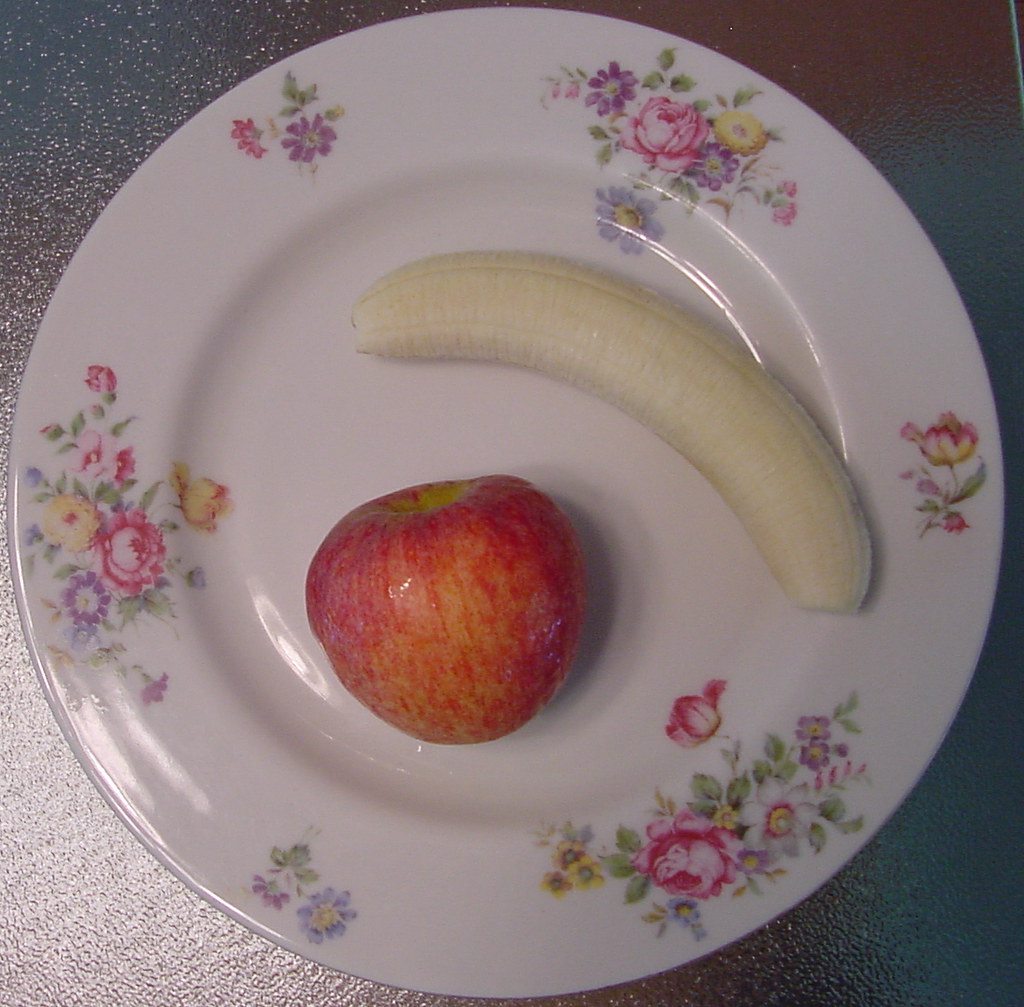This image is a top-down photograph featuring a sophisticated table setting with a striking contrast between dark and light elements. The table is a deep, perhaps black color, providing a stark backdrop for a pristine white plate that appears to be crafted from ceramic or fine china. This elegant plate boasts a delicate floral print, showcasing an array of multicolored flowers. Among them are pink roses, purple blooms, blue flowers, and vibrant yellow daisies, all interspersed with green stems and leaves. The floral arrangement on the plate features three main clusters of flowers and three smaller clusters, each with one or two blossoms.

Resting on this ornate plate are two pieces of fruit: a whole, peeled banana displayed at the top, and an unblemished apple situated below it. The banana, fully peeled but not segmented, lies in its entirety, its smooth texture contrasting with the plate's floral detail. Below the banana, a whole, uncut apple with a red skin tinged with yellow sits without a stem. The apple, casting a shadow, emphasizes its fullness and untouched exterior. The overall composition merges the simplicity of fresh fruit with the intricate elegance of the floral plate, creating a visually appealing and richly detailed scene.